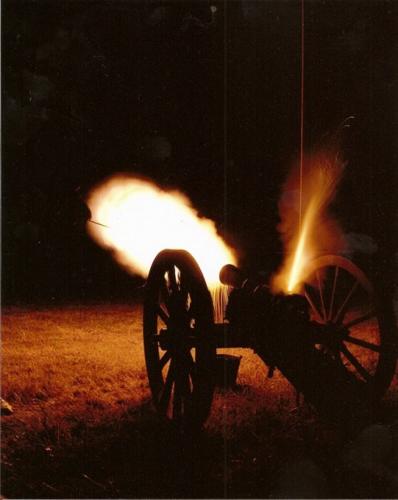The photo captures a night scene of a historic military cannon firing in mid-blast. The large cannon, equipped with two sizable wagon wheels, is positioned in an open grassy area. The darkness enveloping the scene is interrupted only by the dramatic flames erupting from both the front muzzle and the rear ignition point. The illuminated blast casts enough light to reveal a patch of grass in front, providing a stark contrast to the nearly complete blackness that shrouds the background. The faint outlines of two vertical glowing lines in the distance are barely visible amidst the darkness. The striking image also captures a secondary flame off to the right side, likely from the ignition fuse, adding to the dramatic intensity of the scene. The overall lack of visibility makes it impossible to discern what the cannon is aimed at, evoking a sense of historical reenactment where the outcome of the shot remains a mystery.